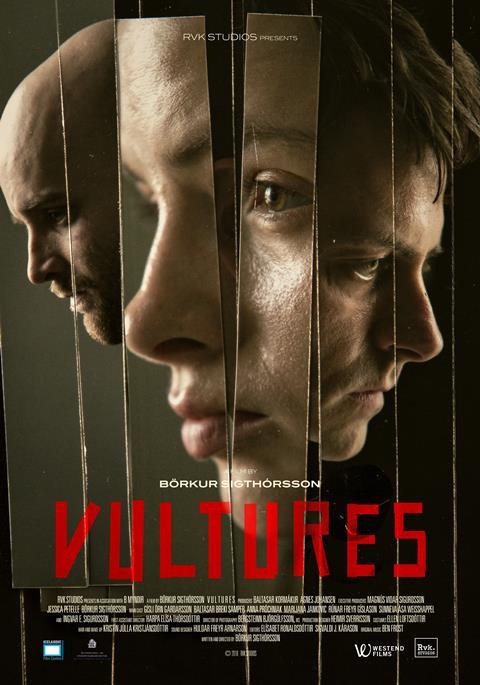This movie poster for "Vultures" is vertically oriented, featuring a fractured, artistic collage of three faces divided into vertical strips. At the top center, it reads "RVK Studio Presents," indicating the production house. Just below, the name "BORKUR SIGTHORSSON" is displayed in all caps white letters, albeit in a smaller font size. Dominating the lower portion of the poster, the title "VULTURES" is printed in bold, all caps red letters. The bottom right corner houses a large "W," representing West End Films.

The artwork shows a bald man with a stern expression and a short mustache and beard on the left, facing sideways. The center strip features a woman's fragmented face with light blue eyes, visually divided between two vertical sections, while the right strip depicts a downcast man with short brown hair looking towards the right. Below the main title, there is a dense block of text including typical Hollywood credits for directors, producers, and actors, although it's too small to read clearly. The overall design indicates a high level of artistic intent and professional production.